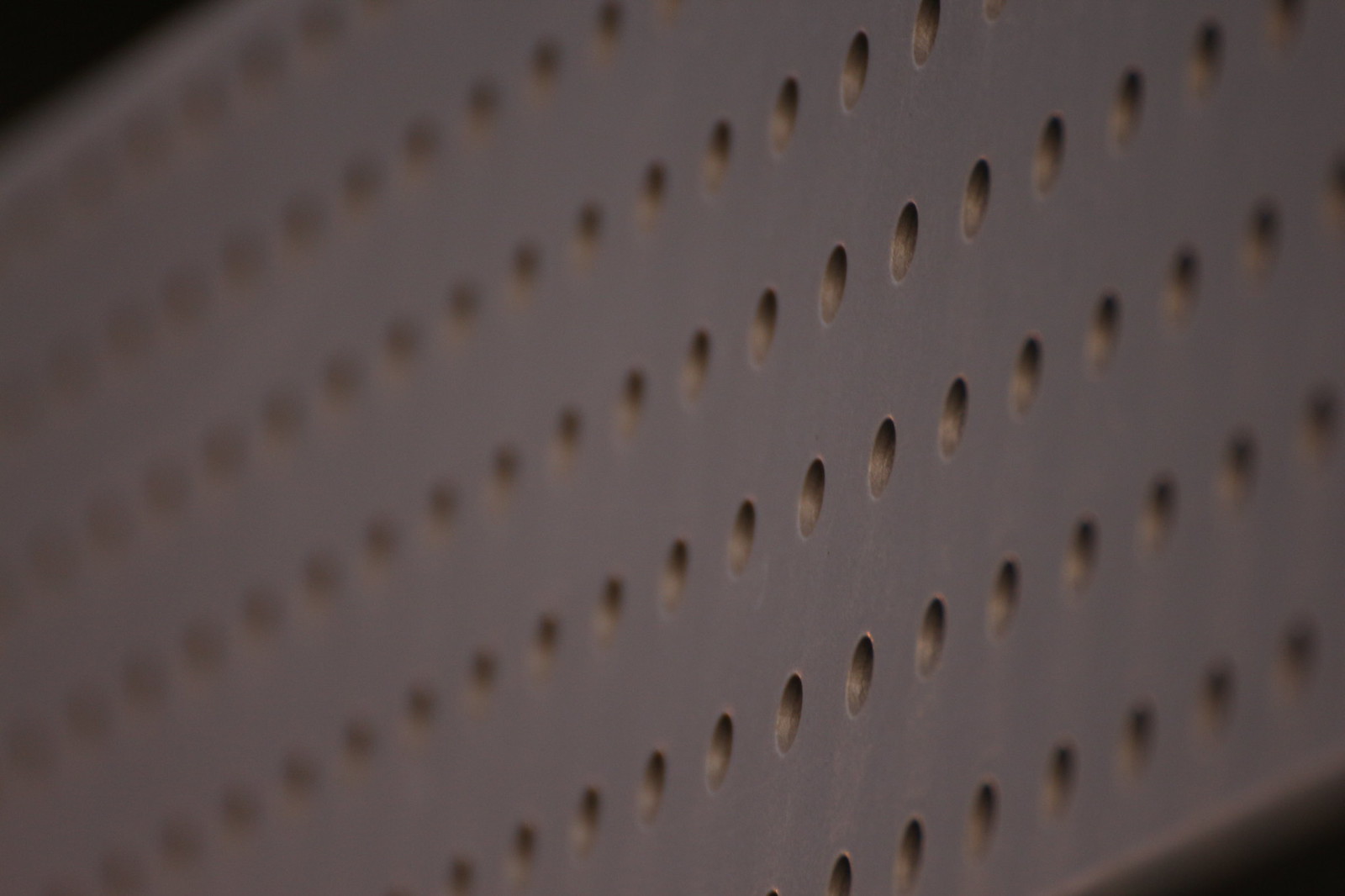This photograph is an extreme close-up of what appears to be a metal pegboard or possibly a vented section of an electronic device, such as the back of a TV. The image is taken at an angle, with the object placed diagonally across the frame, occupying the majority of the photograph. The surface of the pegboard is a grayish-black color, perforated with rows of evenly spaced, symmetrical holes. 

The left side of the image is notably blurry, with the focus gradually sharpening towards the right, although there is still some minor blur on the right edge. This close-up perspective reveals about seven or eight clear rows of holes, with shadows visible inside some of the central holes, adding depth to the photograph. There's a slight presence of dust within the holes, suggesting it might be an older or frequently used item. The image does have a little bit of what seems like plaque or grime on the top left corner and the bottom right.